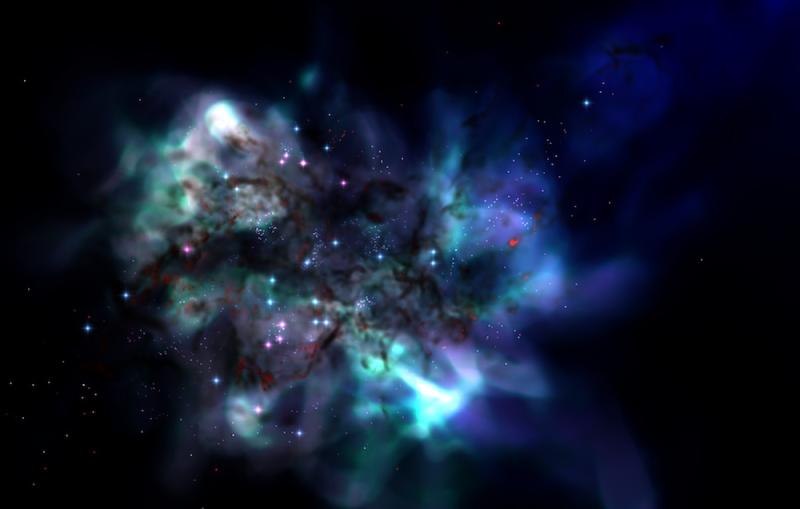This image depicts a mesmerizing cosmic scene likely of a nebula, captured in vivid detail. Dominated by hues of blue, green, and violet, the nebula appears as a swirling mass with a bright central core from which splotches and streaks of dust and gas emanate. The translucent clouds in the nebula show striking contrasts, featuring light blue, emerald green, and white with traces of cherry red that blend seamlessly with the surrounding colors. Delicate, star-like dots—blue and purple—shine through the gaseous clouds, adding depth and intricacy to the composition. The backdrop of the image is the dark, sprawling expanse of deep space, emphasizing the vastness and beauty of the universe and evoking a profound sense of awe and wonder.